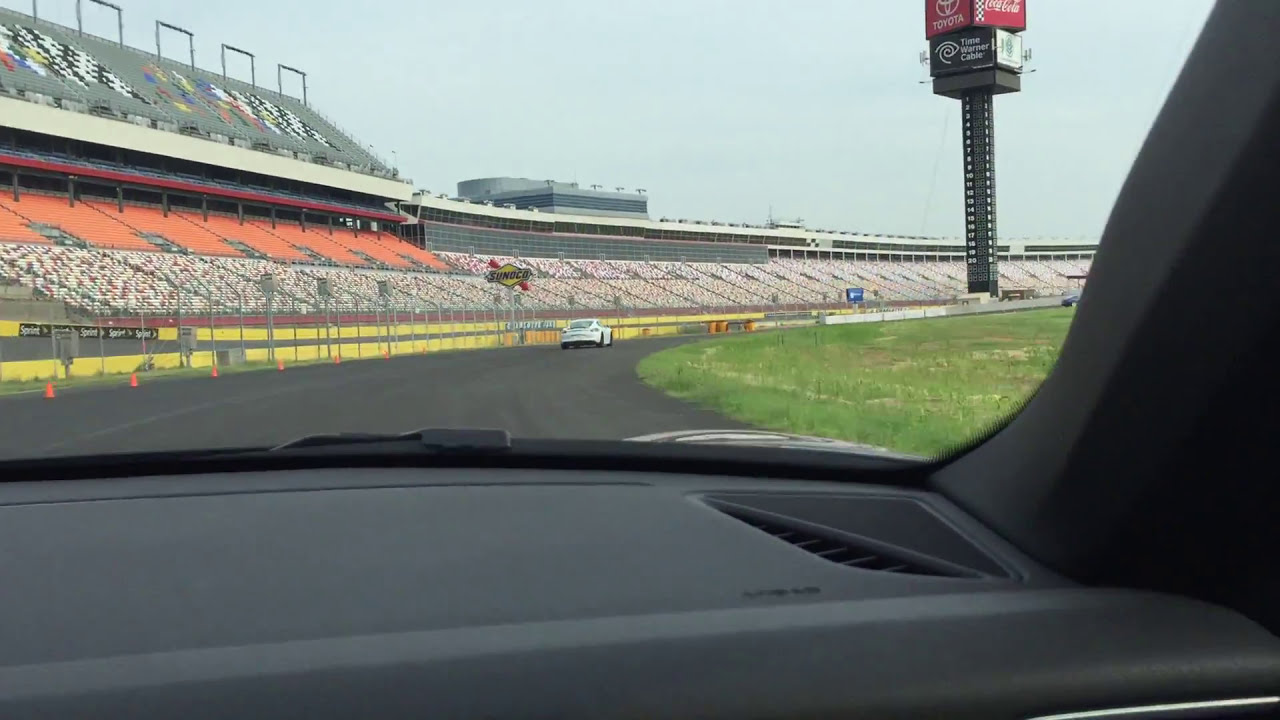This photograph captures a dynamic racetrack scene from the perspective of being inside a car, showcasing the vehicle's charcoal gray dashboard with a visible vent on the right side. The view through the front window reveals a curved, black asphalt racetrack set within a bustling stadium, with a white car prominently featured on the track about 20 to 50 feet ahead. To the right of the track is a grassy field, while the left side is lined with yellow barriers and a large metal fence separating the track from the audience area.

Above the racetrack, the stadium seats—comprised of black, white, and multicolored spots suggesting a crowded audience—arc along the curvature of the track. Dotting the scene are numerous flags and advertisements, including a tall metallic column with red and black advertisement cubes; the red cube displays the Toyota logo, while the black cube bears the name "Time Warner Cable." Further enhancing the commercial ambiance, there is a notable Sunoco sign to the left and a Brawny advertisement in the spectator area. Overhead, a cloudless sky provides the perfect backdrop for this vibrant snapshot of modern racing. The entire setting appears to be from a recent digital racing game simulation, bringing the high-speed thrill vividly to life.